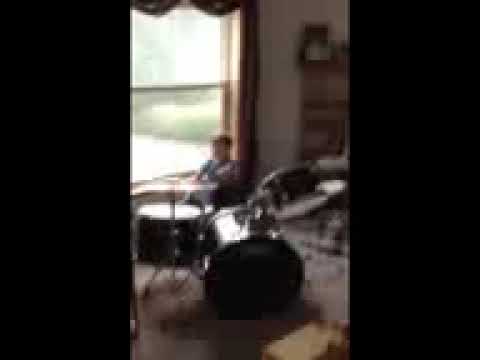This is a fuzzy, pixelated, and out-of-focus image depicting a young boy, approximately five or six years old, standing or sitting off to the left or middle-left of the frame, potentially playing or practicing on a black drum set with silver trim. The boy, with light brown hair, is situated in front of a window, through which light illuminates his head and the drum set. The photo, which appears to have been taken with an older, low-quality camera, showcases the boy amidst four or five drums and a cymbal, arranged both in front of him and scattered around the room. The scene is set within a home, with the backdrop consisting of walls painted in shades of white, beige, and brown, and a shelf visible at the top. The image is further framed by noticeable black borders on both the left and right sides. Overall, the photograph is grainy and lacks detail, making it challenging to discern precise colors and finer elements of the setting.